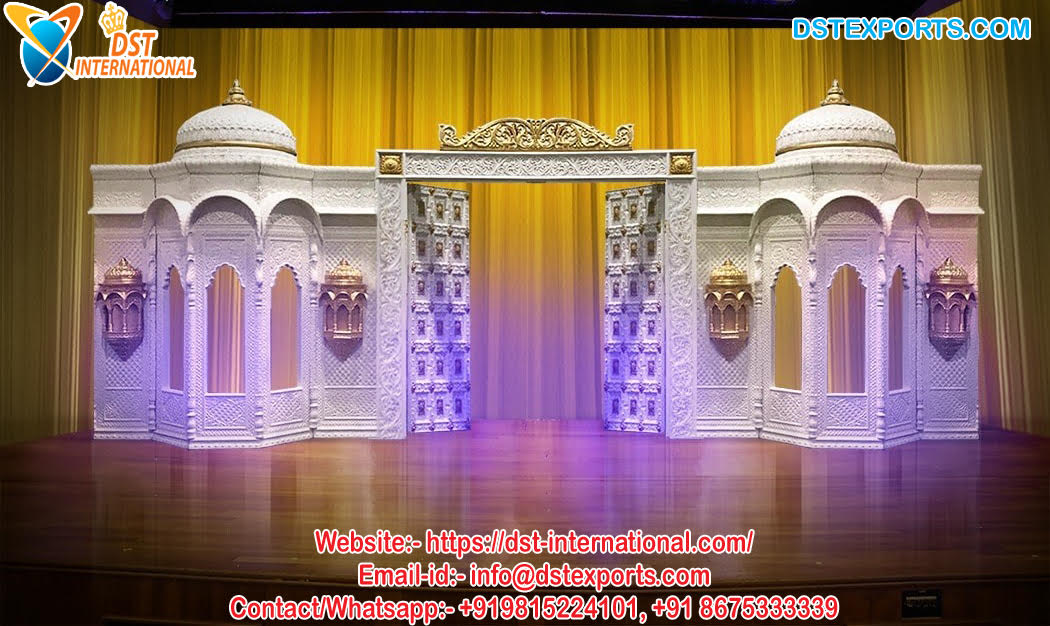This photographic image captures an opulent indoor stage setup reminiscent of Middle Eastern architecture, possibly inspired by iconic Indian structures like the Taj Mahal. The stage features two identical, white marble kiosks with domes topped by metal tips. Each kiosk has three arched bay windows framed in white, flanked by smaller structures mimicking the main design, adorned with ornate golden lanterns. A grand archway and a white-and-gold door with intricate metal framework connect the kiosks. The stage’s backdrop boasts gleaming gold curtains with purple lights reflecting off them, while the floor appears to be polished wood. The entire image is framed by text, including a top-left corner logo for DST International with a blue-shaded globe and orange rings, the website dstexports.com prominently displayed in blue on the upper right, and contact details at the bottom center in orange and white, providing the website URL, email address, and two WhatsApp phone numbers.